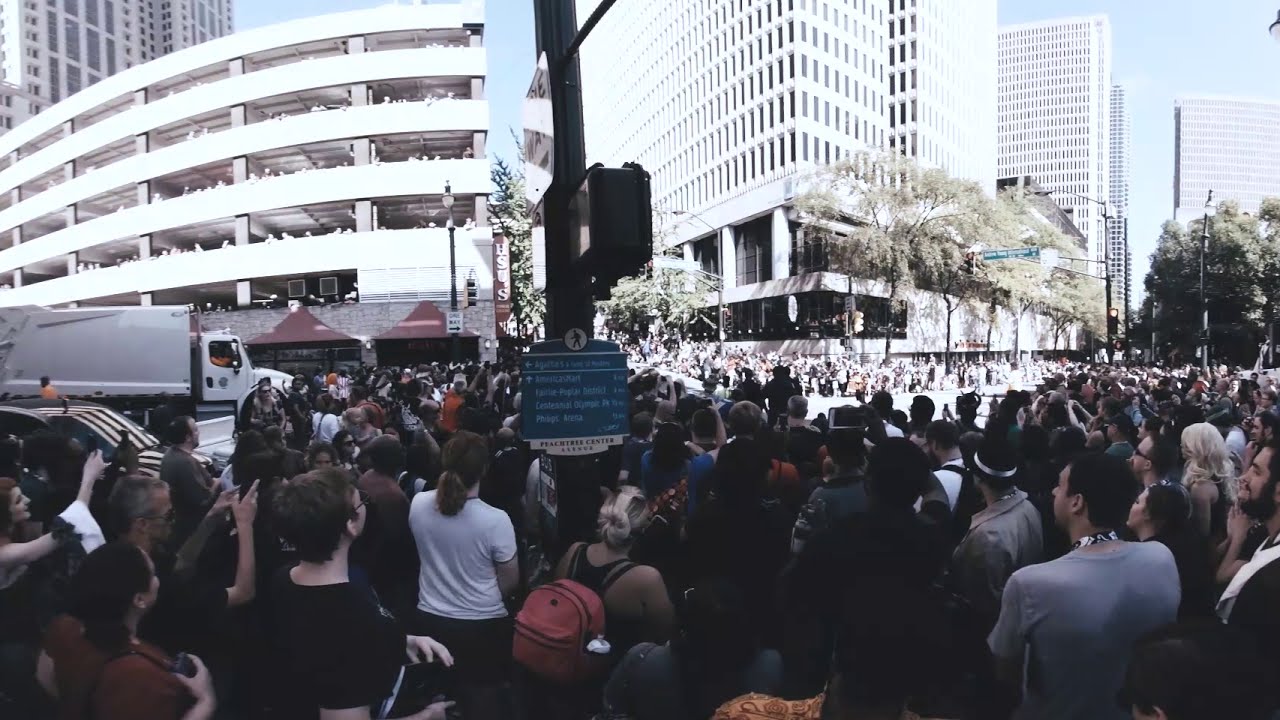This image captures a bustling city street corner filled with a densely packed crowd of hundreds of people, indicating a significant event or gathering. The photo is taken from above, using a fisheye or panoramic lens, and showcases a diverse crowd, many of whom are holding up their smartphones to take pictures. People are gathered on both sides of the street, suggesting they might be waiting for a parade to start or observing an ongoing festivity. Prominently in the middle, there is a black pole with a green pedestrian information sign featuring five lines of white text, though its details are unclear. A white truck appears halted at a traffic signal in the midst of the crowd. On the left side of the frame is a rounded, six-level parking garage with people watching from the upper levels. In the background, towering skyscrapers rise above a treeline, framed by a bright blue daytime sky. The right side also reveals several more tall office buildings, enhancing the urban context of this lively scene.